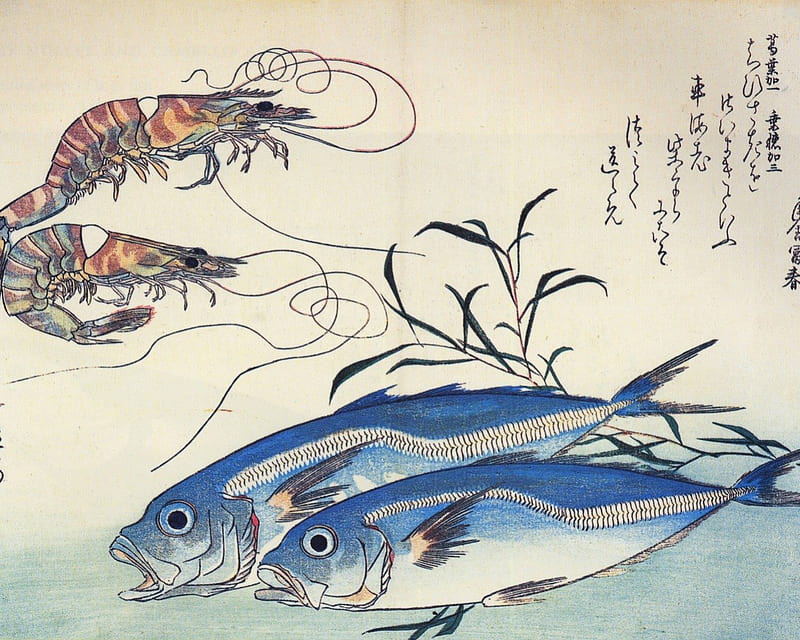This is a detailed color illustration depicting an underwater scene. In the foreground, two blue fish both appear with their mouths agape; their eyes are pale blue with striking dark pupils, and intricate white designs run along their sides. Behind them, a sprig of seaweed adds depth to the composition. In the top left corner, two shrimp are visible. The upper shrimp displays its tail splayed elegantly behind it, while the shrimp below has its tail curved beneath its body. Their notably long antennae twist and wave fluidly through the water. The top right corner of the illustration features Japanese script. The artwork is set against a predominantly white backdrop with subtle blue shading at the bottom, adding to the underwater ambiance. The illustration is devoid of English text and human figures, focusing purely on marine life and its surroundings.